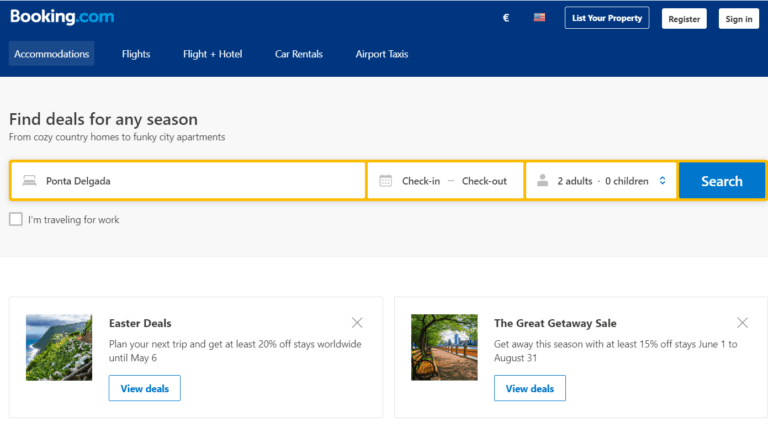**Detailed Descriptive Caption:**

This screenshot captures the homepage of Booking.com, showcasing a well-organized and user-friendly interface. At the top of the page is a distinctive blue banner indicating the user is browsing from the United States, though a Euro symbol is also visible, which may cause some confusion. In the top right corner, users are given options to "List your property," "Register," or "Sign in."

Below the prominent Booking.com logo, various categories are available: "Accommodations," "Flights," "Flight + Hotel," "Car Rentals," and "Airport Taxis." The main part of the page features a large rectangular banner with a welcoming message encouraging users to "Find deals for any season, from cozy country homes to funky city apartments."

Users are prompted to enter their desired location in a search text box, select check-in and check-out dates via a calendar, and specify the number of adults and children for the search. There is a blue "Search" button alongside an option to indicate "I'm traveling for work."

Further down, two promotional boxes are shown. The first highlights "Easter deals," inviting travelers to plan their next trip with discounts of at least 20% off stays worldwide until May 6th, with a "View details" link provided. The second box advertises the "Great Getaway Sale," offering at least 15% off stays from June 1st to August 31st, also with a "View details" link.